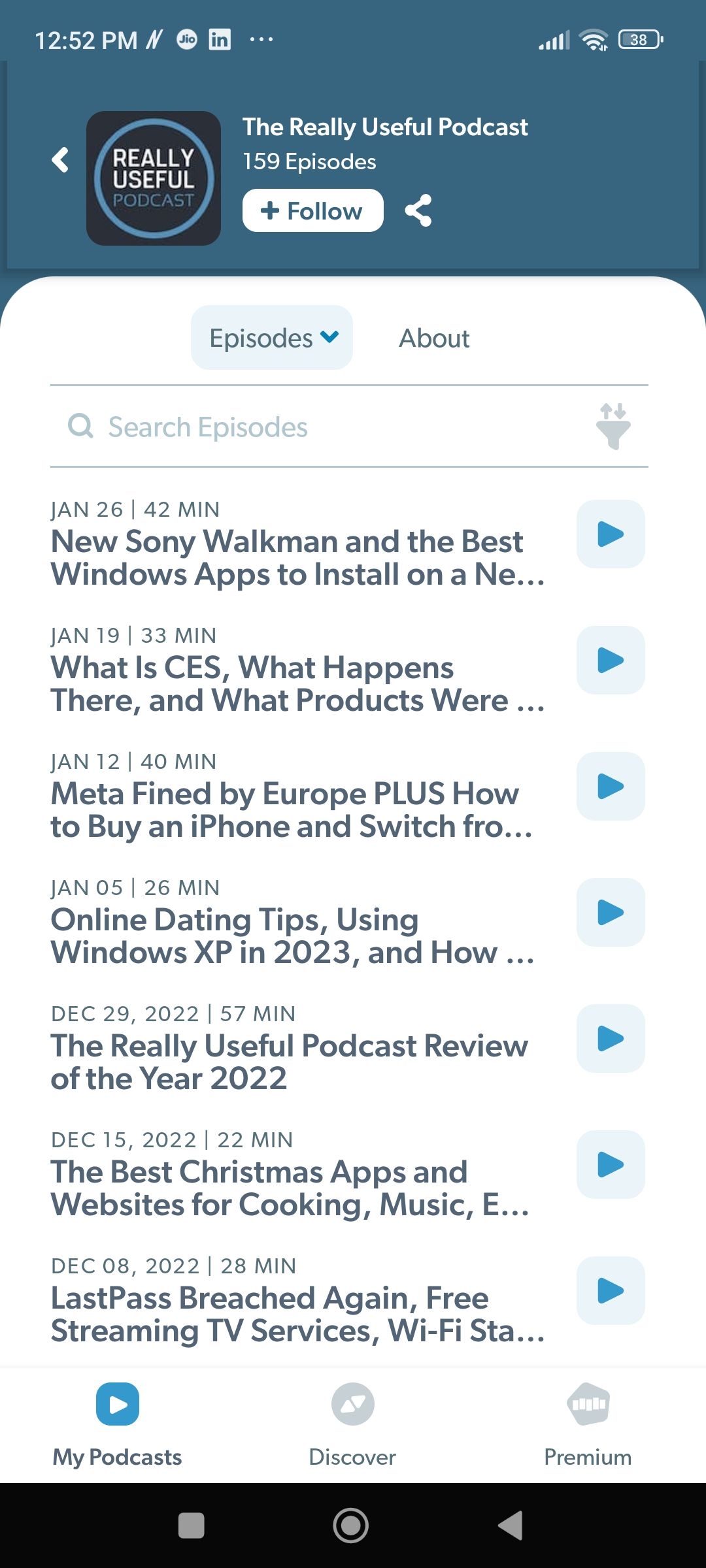This image is a screenshot from the Really Useful podcast page on a mobile application. The header displays "Really Useful Podcast" with a total of 159 episodes available. There's a follow button prominently displayed inside a white circle. The time on the device is shown as 12:52 p.m., and the battery indicator shows either 32% or 38% charge, alongside a connectivity symbol indicating a strong signal with three out of four bars.

The screen is segmented into various sections. At the top, beneath the header, there are tabs labeled "Episodes" (highlighted in a blue box) and "About." The "Episodes" tab has a dropdown menu, and a search bar labeled "Search episodes" is also visible.

Below the search bar, a list of recent podcast episodes is displayed, featuring titles and partial descriptions, along with their release dates:
1. **January 26** - "New Sony Walkman and the Best Windows Apps to Install on a NE..."
2. **January 19** - "What is CES, What Happens There, and What Products Were..."
3. **January 12** - "Meta Fined by Europe Plus, How to Buy an iPhone and Switch From..."
4. **January 5** - "Online Dating Tips Using Windows XP in 2023, and How..."
5. **December 29, 2022** - "The Really Useful Podcast Review of the Year, 2022..."
6. **December 15** - "The Best Christmas Apps and Websites for Cooking, Music, E..."
7. **Last Pass Breached Again, Free Streaming TV Services, Wi-Fi Station..."

At the bottom of the screen, there's a navigation bar with options labeled "My Podcasts," "Discover," and "Premium." This is contained within a black bar that also features icons: a square, a home button, and a left-facing arrow.

The overall layout and details suggest a comprehensive and user-friendly interface, allowing listeners to easily navigate and explore the episodes of the Really Useful podcast.